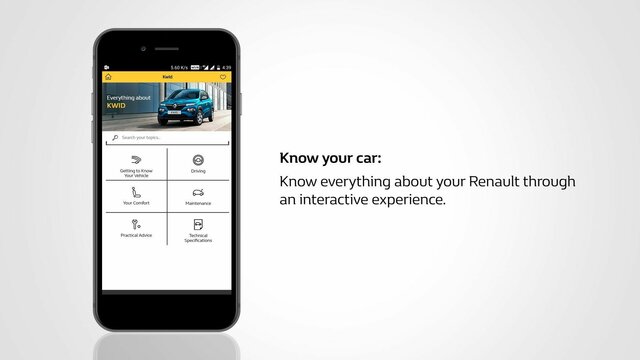The image is a display ad featuring a rectangular layout that is wider than it is tall. The background is a subtle light gray shade. Positioned centrally is the headline in bold font, stating "Know Your Car." Below this headline, there is a subtext that reads, "Know everything about your Renault through an interactive experience."

To the left of this text, there is an illustration of a black-framed smartphone casting a medium shadow at the bottom. The smartphone appears to showcase the digital interface associated with Renault automobiles. The top of the smartphone screen displays a yellow border, beneath which is an aquamarine green photo of a Renault car parked beside some storefronts. 

Directly below the car image is a white background section featuring a search box at the top. The remaining area of the screen is divided into six sections, each accompanied by icons, although the font size is too small to decipher the exact labels. This probably indicates that the digital interface is more likely a website rather than an app.